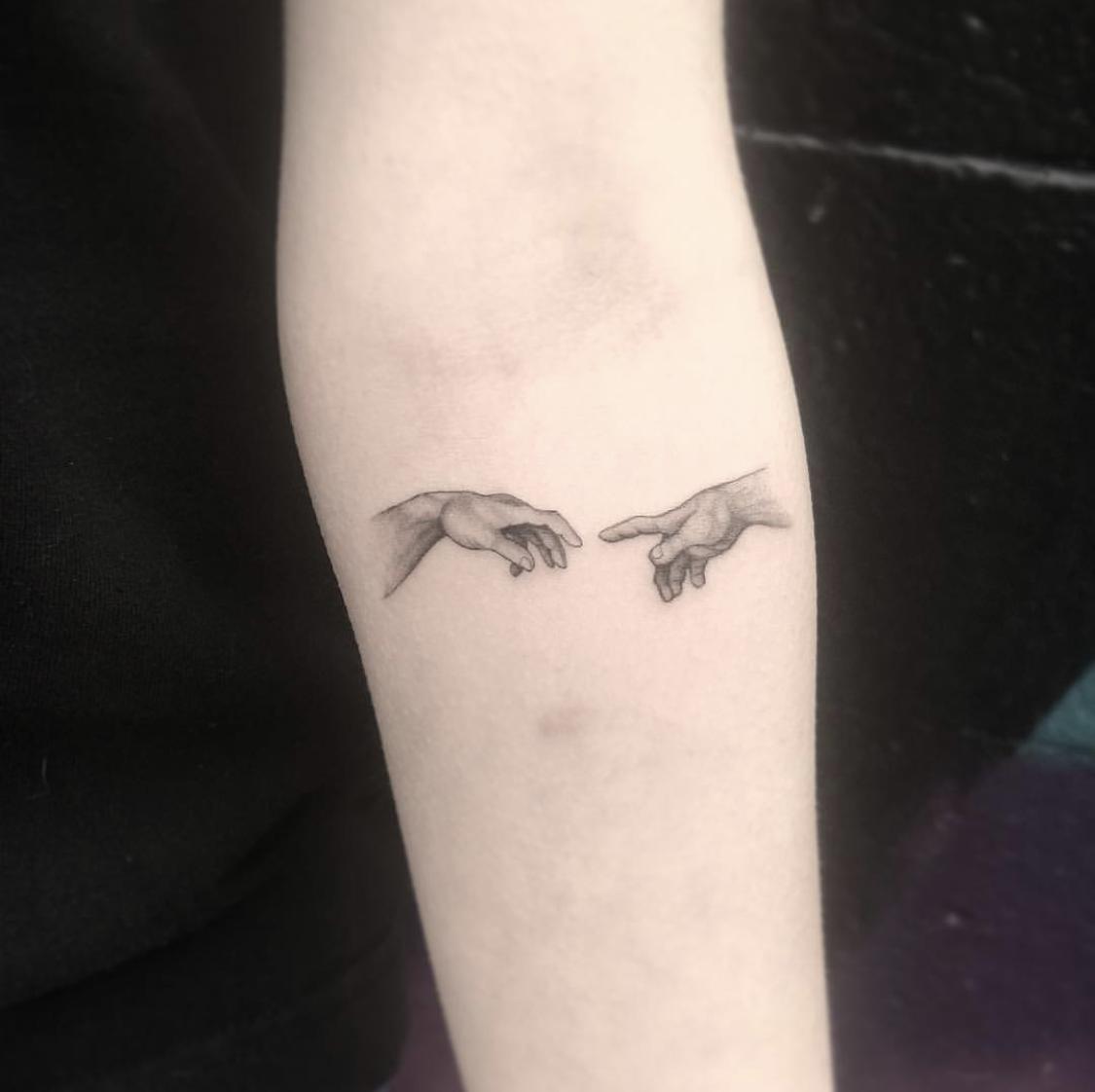The photograph features the inner forearm of a white individual, prominently displaying a detailed grayscale tattoo. The tattoo is a realistic depiction inspired by Michelangelo’s iconic painting from the Sistine Chapel, showing the hand of God reaching out to the hand of Adam. Positioned just below the elbow crease, the left hand extends towards the right hand, with the latter's index finger pointing back, capturing a timeless moment of connection. The dark, unfocused background enhances the focus on the intricately designed tattoo, providing a stark contrast that highlights the artistic detail and the curvature of the forearm.